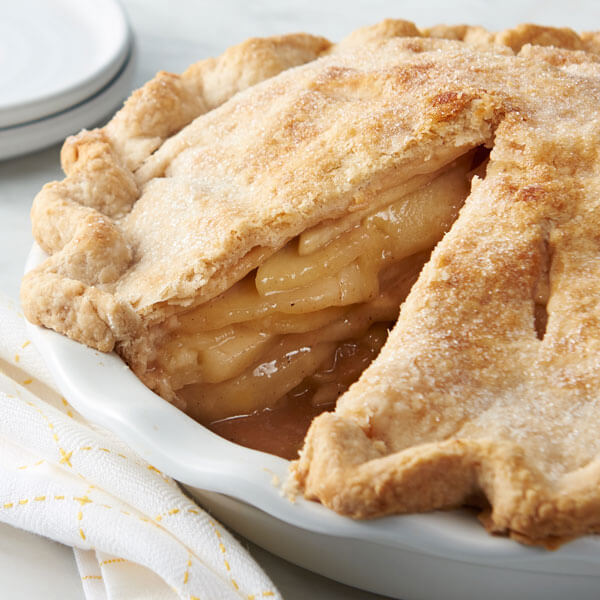This detailed image captures a beautifully homemade apple pie, featured in a white ceramic pie plate, likely from a Finnish food blog. The golden-brown crust is thick, flaky, and meticulously braided around the rim, showcasing impressive baking skills. A generous dusting of sugar crystals on top appears caramelized to perfection, enhancing its crisp texture. Visible specks of cinnamon and possibly vanilla add a touch of spice to the layers of moist apples within. A small slice has been cut from the pie, revealing the juicy, well-layered apples inside. The pie sits on a pristine white marble table, accompanied by a couple of white plates and a cream napkin adorned with yellow embroidery, completing the cozy, inviting presentation.